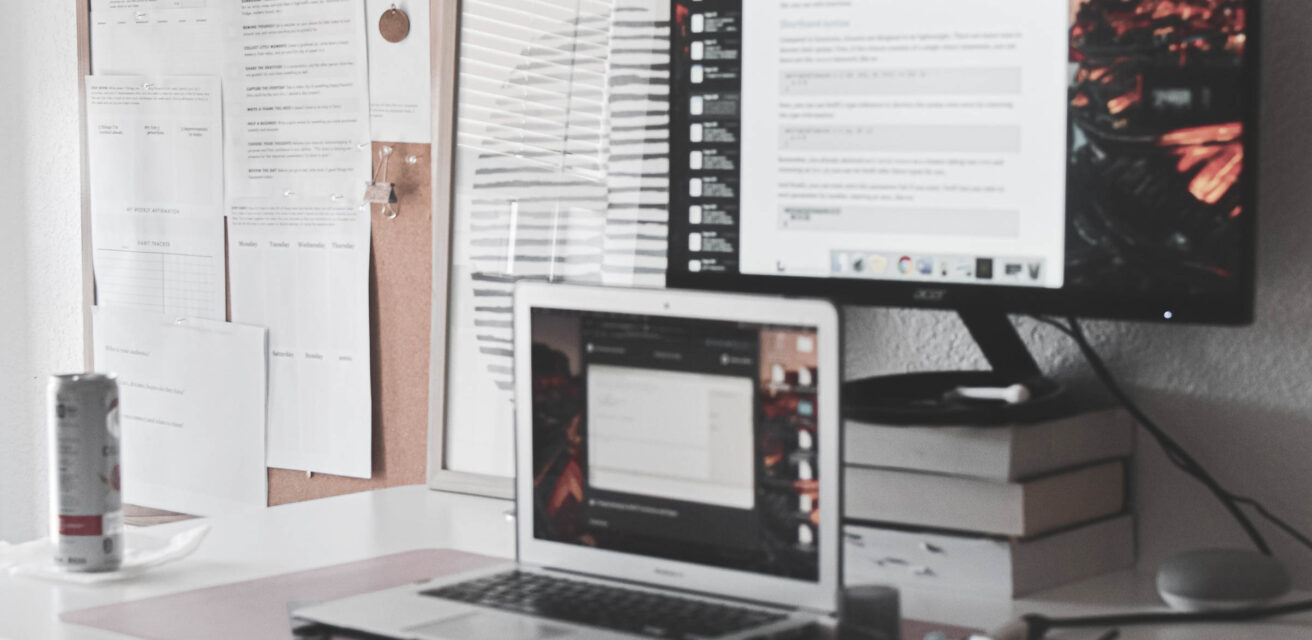The image depicts a cluttered desk setup taken in a poorly focused, horizontally rectangular full-color photograph. Central to the composition is an open gray laptop displaying an indistinct website or program, situated on a white, likely plastic or formica, table. Directly behind the laptop, an LED computer monitor is perched atop three thick books, displaying what appears to be a split-screen view with a Word document on the left and an orange-toned mosaic illustration on the right.

To the left of the desk sits a blurry silver aluminum can, likely a Celsius energy drink, adding a touch of casual disarray. Further to the left, a wall-mounted cork board draped in a pinkish hue is densely covered with several pinned white papers, contributing to the workspace's chaotic feel. On the right side of the desk, a small, grey Google Home device adds a modern tech touch. The overall photograph captures an everyday desk environment cluttered with work materials and personal items, portrayed in a soft, unfocused blur.